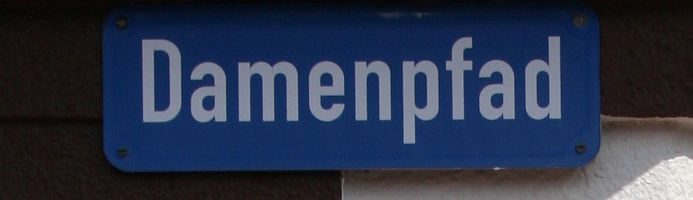The image portrays a blue street sign with white letters spelling "Damenpfad." The sign has a rectangular shape with curved edges and appears tilted 270 degrees, oriented vertically. The capital "D" is closest to the bottom of the image, with the rest of the letters stacking upward, requiring you to tilt your head left to read it properly. The sign is affixed to a darker, textured background, possibly with black metal and a white rectangular base or fastener at the bottom, which appears chalky or painted. There are screws located in the lower right and lower left corners of the sign. The overall background is mostly dark, but the upper right quadrant is lighter, possibly brown, adding contrast to the blue sign.